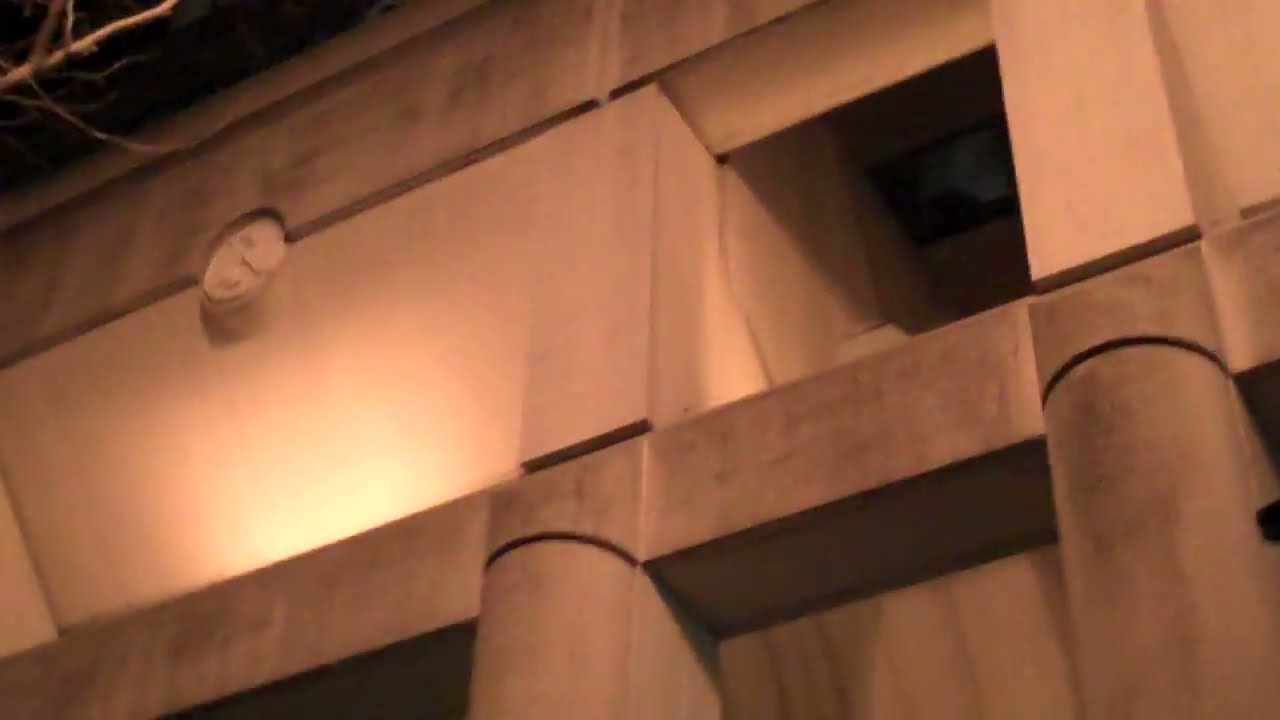This image is a blurred, nighttime color photograph, captured from the perspective of a sidewalk looking up between towering high-rise buildings. The scene is dark, bathed in varying shades of brown and deep amber tones. Dominating the middle right of the image is a three-globed street lamp emitting a golden-orange glow. Scattered lights twinkle from the windows of apartments on the right and an office building on the left, adding sporadic illumination to the otherwise dim setting. In the foreground, partially obscured, is the silhouette of a man clad in black, possibly a police officer, viewed from behind with a large belt adorned with equipment around his waist. The image is tilted upwards, revealing the tops of some trees nestled between the buildings, though they are barely discernible in the dark. The overall effect is a moody, almost surreal urban landscape, barely defined by its dim lights and blurred structures.